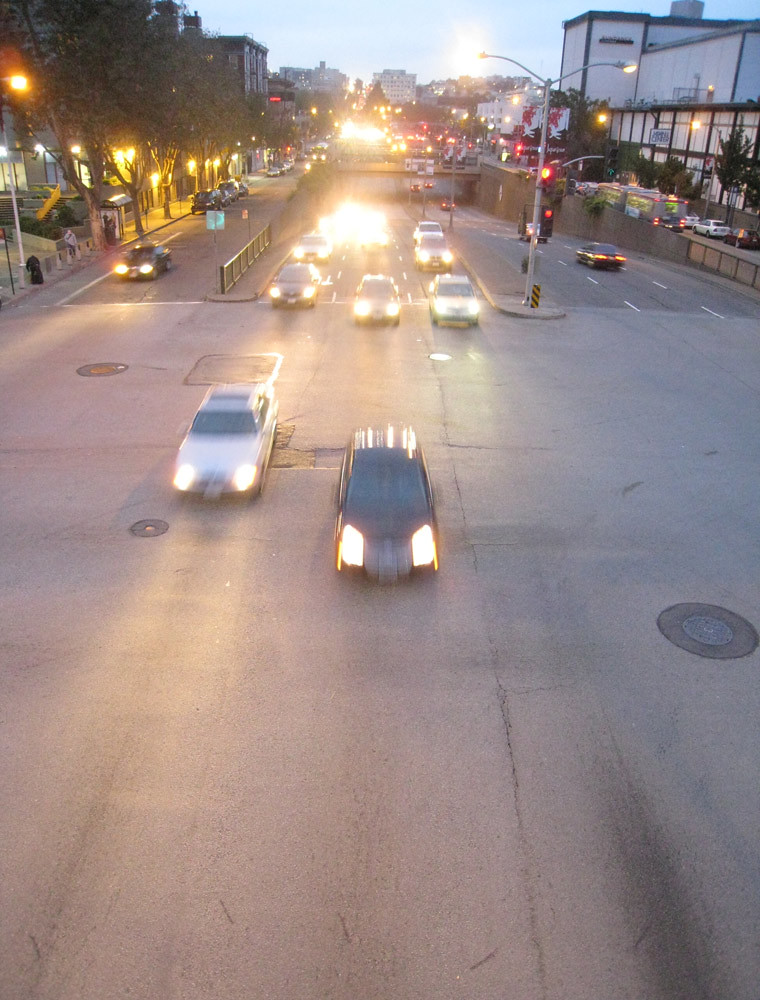The photograph depicts a bustling urban scene as evening descends, likely set in a downtown area. The image captures a busy intersection with a mix of incoming and outgoing traffic, showing a variety of brightly lit cars in colors like white, black, and gray. The streets are lined with buildings that include businesses, apartments, and other structures, while trees dot the sidewalks. As dusk settles in, the sky is growing darker and the streetlights are illuminated, casting a glow over the area. Traffic lights show red, green, and yellow signals, and a "don't walk" sign is visible. Despite the slight blur, the photo clearly shows cars navigating both sides of the road, some appearing to be coming from under a bridge. There are a few pedestrians walking along the street, emphasizing the lively nature of this city environment during what seems to be rush hour.